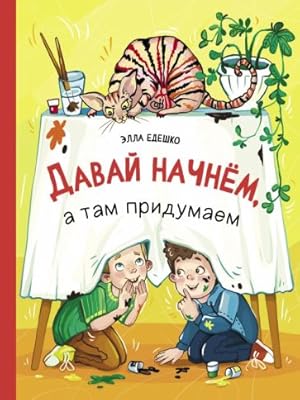The image is a rectangular book cover for a children's book. The spine features a vertical red stripe on the left side, while the main cover showcases a vivid scene. The background consists of a yellow wall transitioning to a brown floor. At the center, there's a round table draped with a white tablecloth adorned with non-English symbols, including an odd-shaped A, backward N, and E with two dots above it. The text reads A-A-B-A backward N H-A-Y-H-E-M, followed by three black words: A, TAM, and another with symbols.

Beneath the tablecloth, two children are playfully hiding and laughing, one signaling 'shh' with a finger to his mouth. One child wears a green top, brown pants, and yellow sneakers, while the other dons an all-blue outfit with orange sneakers. Surrounding them is spilled paint. 

On the table above, a striped cat with a beige body, black and red stripes, and large ears sits confidently, its tail poised upwards. Nearby, there's a glass holding paintbrushes and a white planter with a thriving plant. The entire scene brims with a playful and mischievous atmosphere.